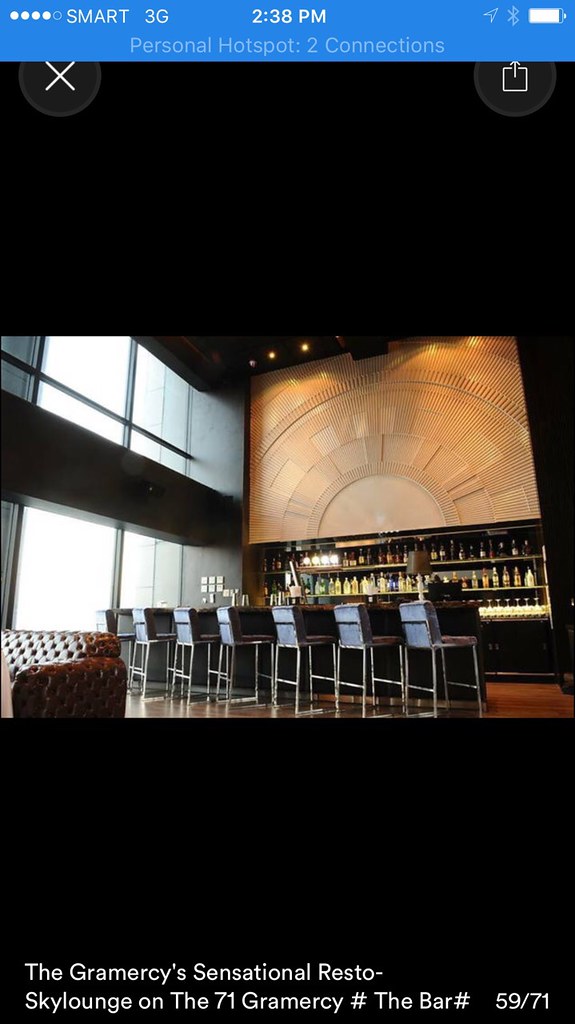The image is a screenshot taken from a phone, marked by a blue bar at the top that states "Smart 3G 2:38 PM" along with the reception indicator and battery symbol. The top bar also indicates a personal hotspot with two connections. The primary focus is a photo of a bar located in the middle third of the screen, framed by black horizontal bars at the top and bottom, with white text at the bottom reading, "The Gramercy's Sensational Resto Skyline Sky Lounge on the 71 Gramercy #thebar," and a photo count of "59 out of 71."

The bar itself is modern yet simple, with dark, wood-topped black counters and gray chairs lining the front. Behind the bar, there’s a striking Art Deco stone-like sun carving. Bright windows with black borders are visible on the left side of the image, while a polka-dotted leather couch sits prominently in the foreground. Along the back wall, rows of shelves hold an assortment of bottles, typical of an upscale, well-stocked bar. Overall, the decor leans towards a darker, elegant motif, creating a sophisticated atmosphere.